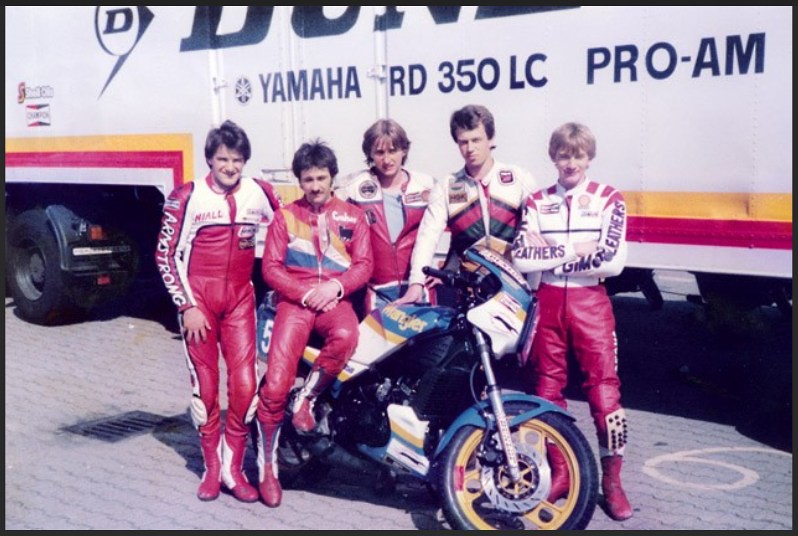This vintage photo, likely from the 1980s, features five men dressed in red and white bodysuits, standing and sitting around a motorcycle. The motorcycle itself is a Yamaha RD350 LC Pro-Am, decorated in blue, white, and gold. The group appears to be part of a motorcycle gang or club. They are positioned on a tiled concrete pavement, and behind them is a large white four-wheeler truck adorned with yellow and red stripes along the bottom. The truck prominently displays the Yamaha brand, suggesting it might be associated with the motorcycle in the image.